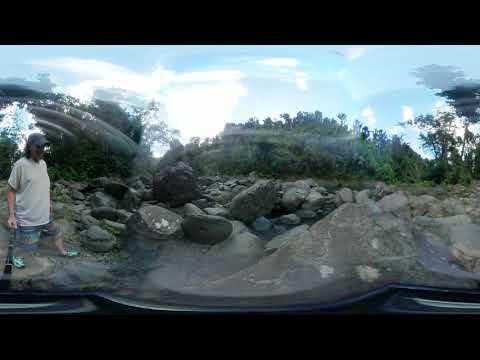A man with a long beard, wearing a grey cap, white short-sleeved t-shirt, blue shorts, and blue shoes, is captured walking in front of a slope filled with large, round stones and boulders of varying sizes. He is holding a black and grey telescopic selfie stick. The background features a line of tall green trees that extend up a low hillside on the horizon. The sky above is light blue adorned with streaky white clouds. The image appears to have been taken through a vehicle's windshield, as indicated by blurry reflections and black bars at the top and bottom of the photo.